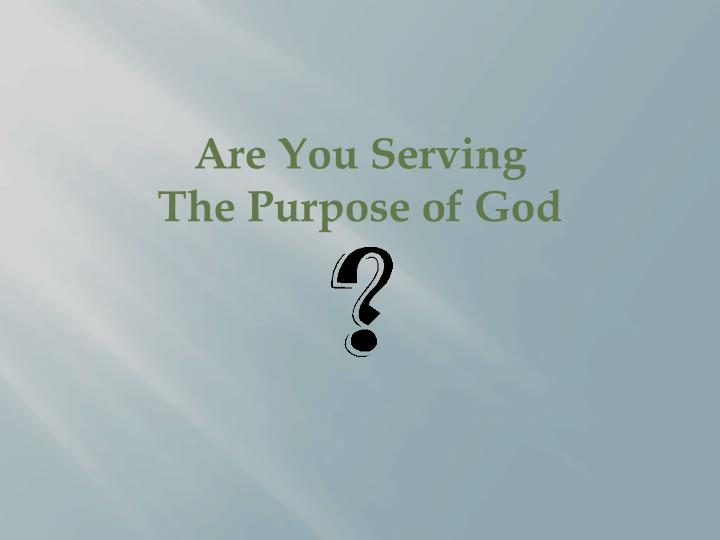This promotional religious image is rectangular, set against a gradient blue background that transitions from dark blue in the bottom right corner to light blue and white in the top left, as if illuminated by beams of sunlight. The central focus of the image is text in an army green, simple font that asks, "Are you serving the purpose of God?" Below this text is a detailed black question mark, which features a slight border along its left edge to give it a 3D effect. The colors present in the image are predominantly blue, white, gray, black, and green, and the design exudes a spiritual and reflective ambiance suitable for use on a webpage, social media board, or as a slide in a presentation.